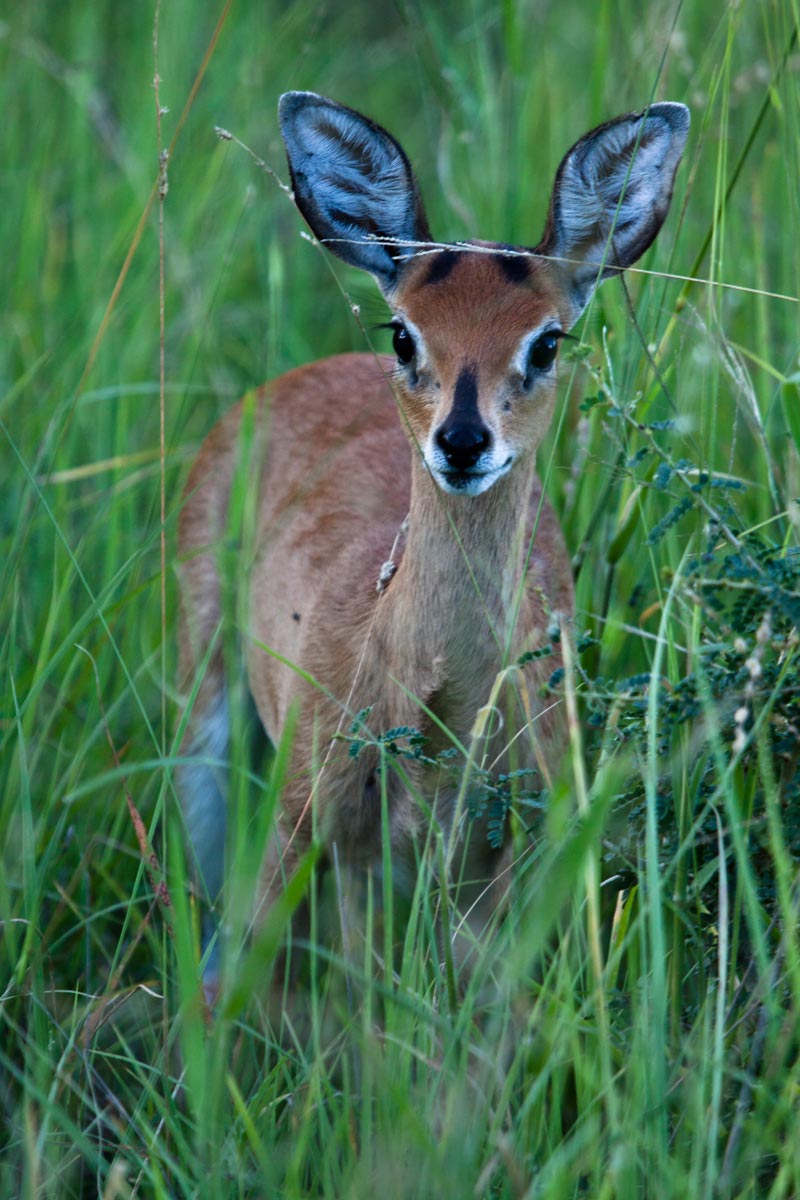This full-color outdoor photograph captures a young fawn standing amidst tall, green grass. The fawn is fawn-colored with some black spots and has striking features including very large black eyes rimmed with white, a black nose, and a white muzzle. Its exceptionally large ears, mottled in color with white fur on the inside, stand prominently from its head. The image is sharply focused on the face of the fawn, highlighting its youthful and innocent appearance. While most of the grass in the foreground is out of focus, adding depth to the scene, a subtle shade of blue in the background adds a calming ambiance to the nature shot. The fawn appears to be staring straight ahead, perhaps curious and unaware of its observer.